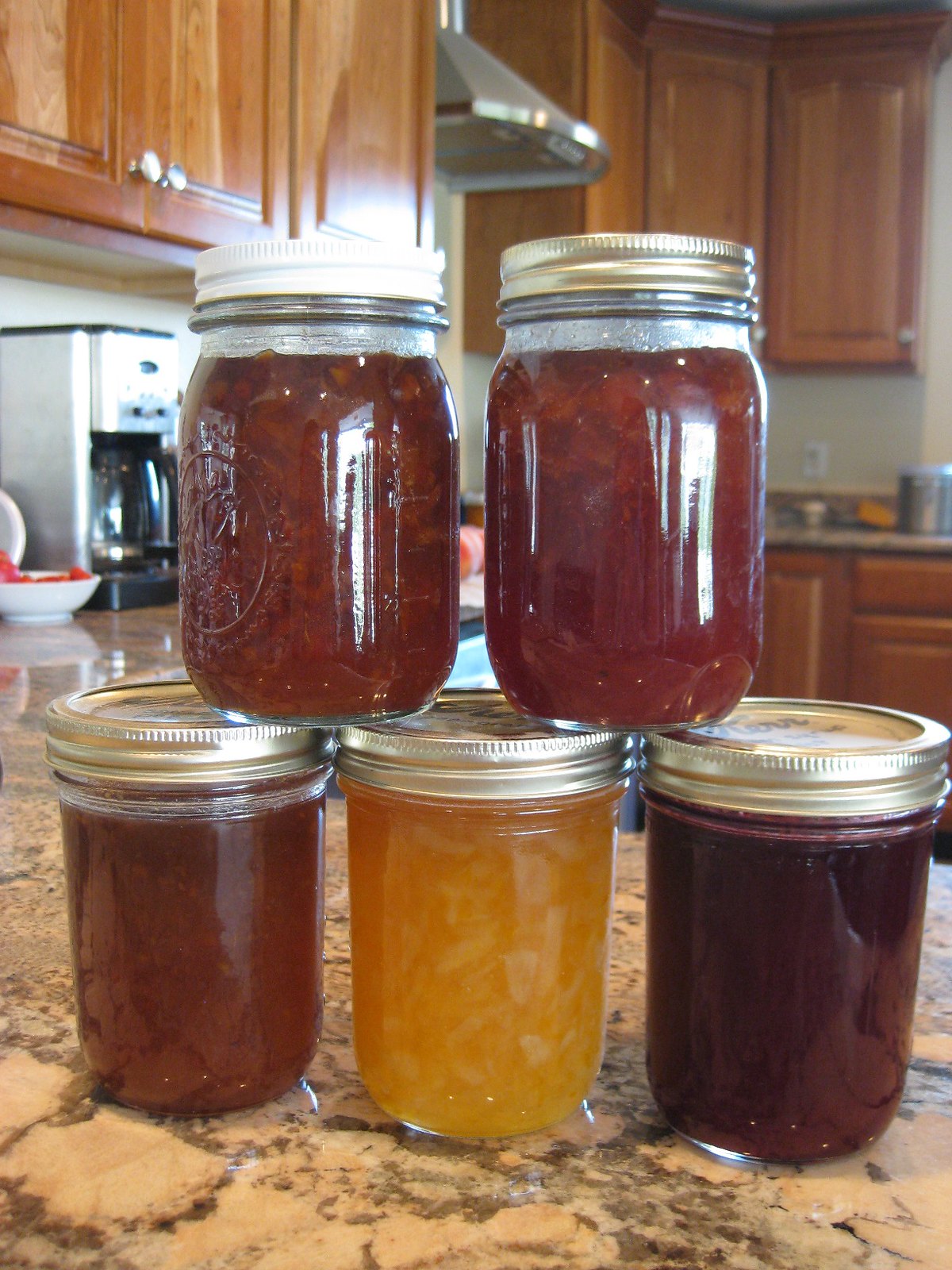In this detailed portrait-oriented photograph, taken inside a home kitchen, we see an artfully arranged stack of five glass jars containing home preserves on a shiny granite countertop. The jars form a pyramid-like structure, with three jars at the bottom row touching each other, and two smaller, slightly conical jars stacked above where the bottom jars meet. The jars, which lack labels, feature a variety of contents - the bottom row includes two uniform dark red preserves on the left and right, and a mustard yellow preserve, possibly marmalade, in the center. The top-row jars are reddish with visible chunks, hinting at a different type of jelly preserve.

The jars themselves are adorned with screw-on lids; four are silver, while the top left jar has a white metal lid. The countertop, showcasing a glossy light beige finish with heavy dark brown striations, adds elegance to the display.

In the background, we can see medium-brown cabinetry with silver handles, typically made from a budget-conscious wood material. A large family-sized coffee maker is placed to the back left of the preserve jars, alongside a white bowl filled with red contents. Other kitchen details include a visible electrical outlet with things plugged into it, and additional objects scattered across the counter, complementing the functional yet homely setting.